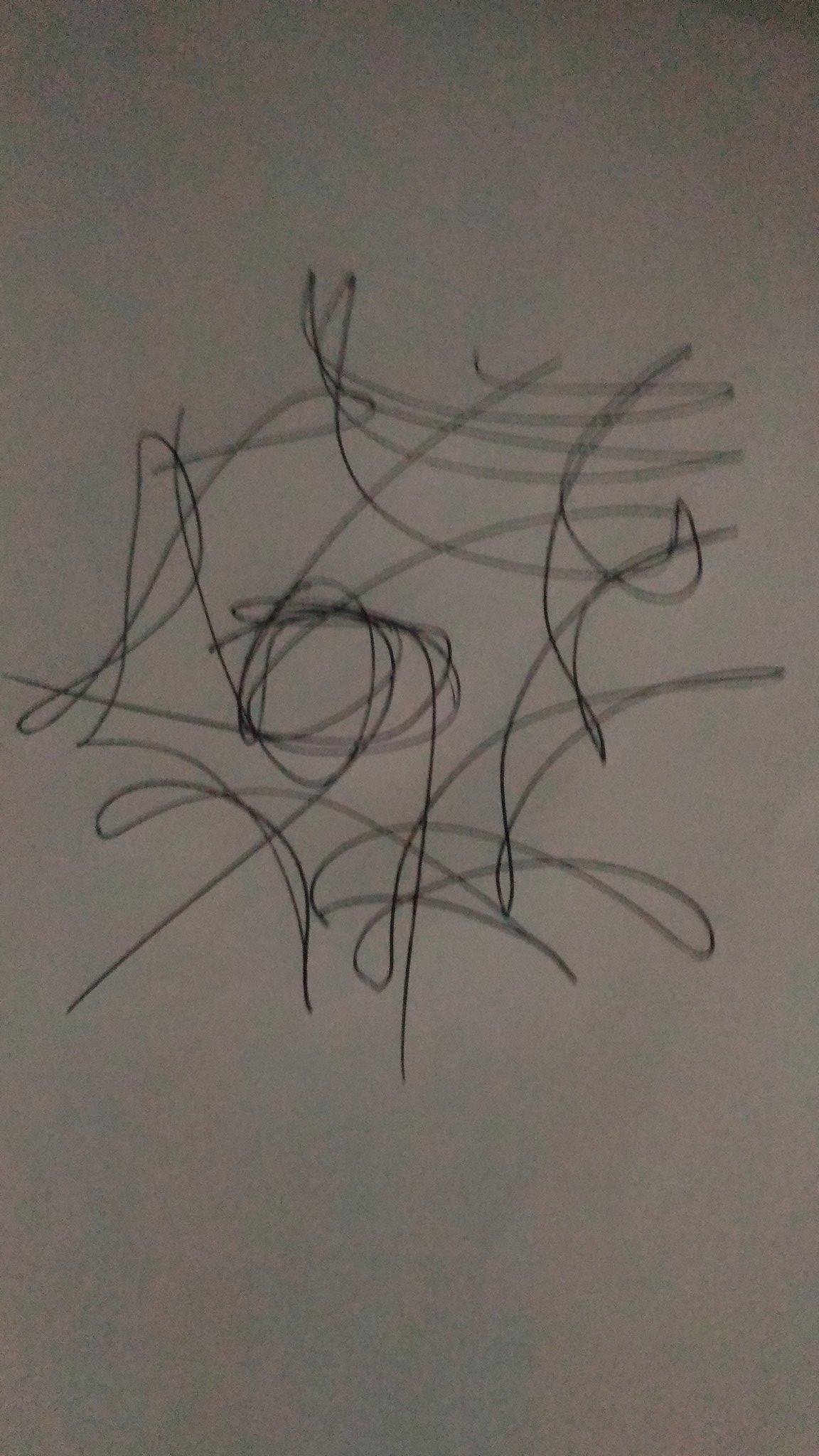This abstract black ink drawing on gray paper features a central circular scribble from which lines radiate outward in a star-like or floral pattern. In the center, the dense ink forms a textured circle, giving an illusion of depth. Radiating outward, the lines extend to the edges of the paper, creating a dynamic composition. At the top, three prominent points stand out with additional lateral lines between them, adding a sense of solidity. The sides each feature a lateral line extending from the center, while the bottom displays about five points, further enhancing the floral or star motif. The entire drawing maintains a monochromatic palette, devoid of any text, focusing purely on the intricate interplay of black lines against the gray background. The overall effect is an engaging, flat composition punctuated by the central circular form and radiating linear elements.